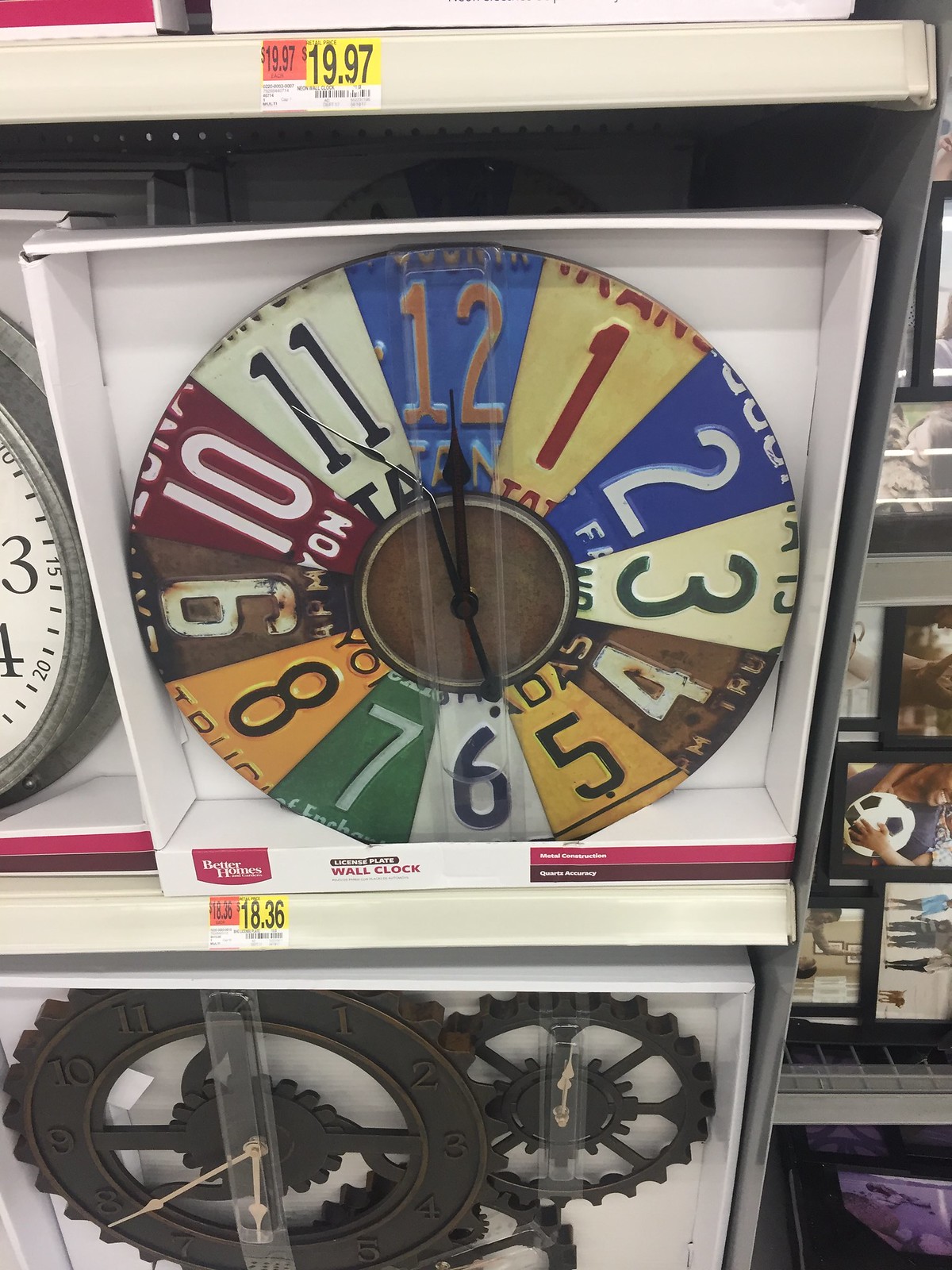This vertical rectangular photograph captures a retail store shelf, likely in a Walmart, showcasing a creatively designed wall clock among other items. The main clock, prominently displayed in a white cardboard box with "Wall Clock" printed in red capital letters on the bottom ledge, consists of segments of variously colored license plates forming a circular pattern for numbers 1 through 12. The license plates show the numbers in distinct colors: 12 (blue with orange), 1 (off-white with red), 2 (dark blue with white), 3 (off-white with green), 4 (brown with white), 5 (orange with navy blue), 6 (white with blue), 7 (green with gray), 8 (orange with blue, hinting at New York with bits of ‘Y’ and ‘O’ visible), 9 (brown with white), 10 (crimson with white), and 11 (off-white with navy). The clock hands are black.

Above the clock, two vertical rectangular price signs display "1997" – one in black writing on a red background and the other in larger black writing on a yellow background, each with unreadable white text underneath. 

Below the license plate clock, another shelf holds a second boxed clock designed with interconnected cogs. This clock features a bronze central gear with numerals and light-colored hour and minute hands, alongside smaller accompaniment gears.

To the right of the license plate clock, the shelf displays picture frames segmented for multiple photos. Visible within the frames is an image of a person holding a soccer ball with their left arm. The price tag on the shelf reads $18.36.